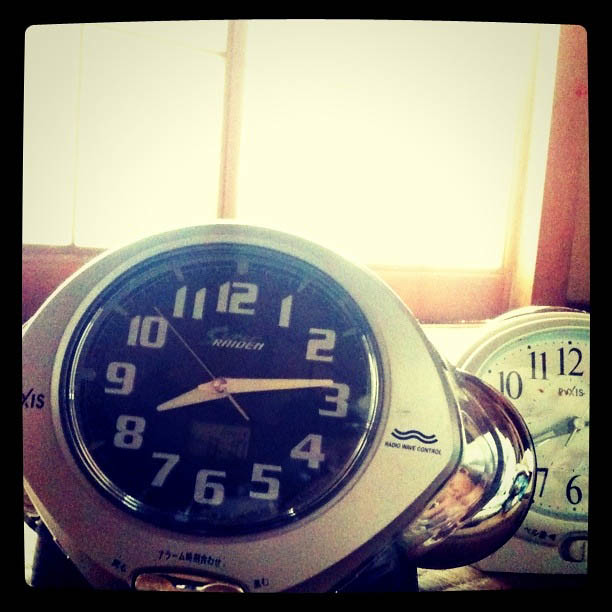The image is a grainy, sepia-toned photograph with a square shape and black border, giving it a vintage feel. It's taken in front of a large window with sheer curtains, allowing bright sunlight to flood in. The window is framed with wood paneling on the right and bottom. In the foreground, two clocks are prominently featured. The larger clock on the left boasts a silver frame, possibly stainless steel or plastic, and has a black face with white numbers and hands. The face displays the brand name "Roden" or possibly "Raiden" below the 12 o'clock position. This clock also has indistinct writing at the bottom and to the sides, with visible words like "Radio Wave Control" accompanied by two blue, wavy lines resembling a river. The time is set to 8:15. To the right of this clock is another, smaller clock with a white face and black numbers. Positioned behind the main clock and to its right, it adds depth to the composition. Additionally, a reflective glass dish on the right side of the main clock captures the faint reflection of two figures, further enriching the scene.